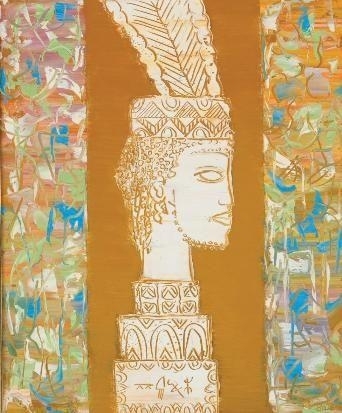The painting presents an abstract depiction of an Indian head drawn centrally on a horizontal brown strip. The head, accentuated in white, features a feathered cap and is in a side profile looking to the right. Below the head, three tiered, block-like structures resemble a layered cake, suggesting the neck and the beginnings of the body. Flanking the head on both sides is a vibrant and chaotic mix of colors including green, blue, brown, orange, purple, pink, and teal, forming a floral-like print that adds to the abstract, playful nature of the artwork. The piece is distinctive for its abstract, almost crude portrayal, blending a detailed central figure with a colorful, seemingly random pattern on either side.